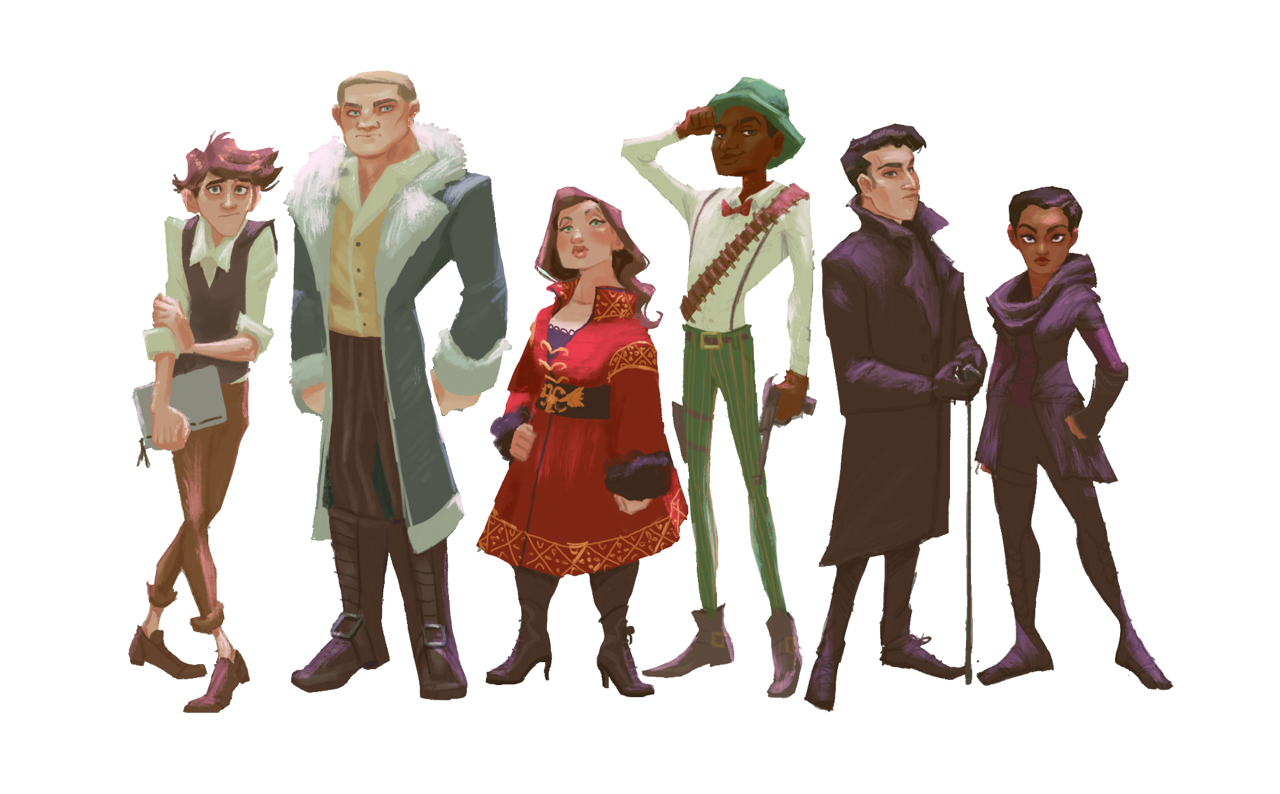The image depicts a vividly detailed, cartoonish group of six characters dressed in historical attire, suggestive of a bygone era. Starting from the left, the first character is a man with reddish hair, wearing a green shirt with rolled-up sleeves, a dark brown vest, light brown pants rolled to the thigh, and brown boots; he is holding a notebook. Next to him is a tall, lean man with dark brown and light brown striped pants, a yellow shirt, and a green fur-lined coat paired with brown boots. The third character is a shorter woman with red hair, dressed in a long red dress and black boots. Standing fourth is another tall man, notable for his green hat, white shirt, green pants, and brown boots. The fifth character is a man in a long, dark-colored overcoat, black pants, and black boots. Lastly, there is a black woman, dressed similarly in a shorter dark-colored coat, dark pants, and matching shoes. All characters stand against a white background, showcasing detailed and distinct attire reflective of clothing from hundreds of years ago.